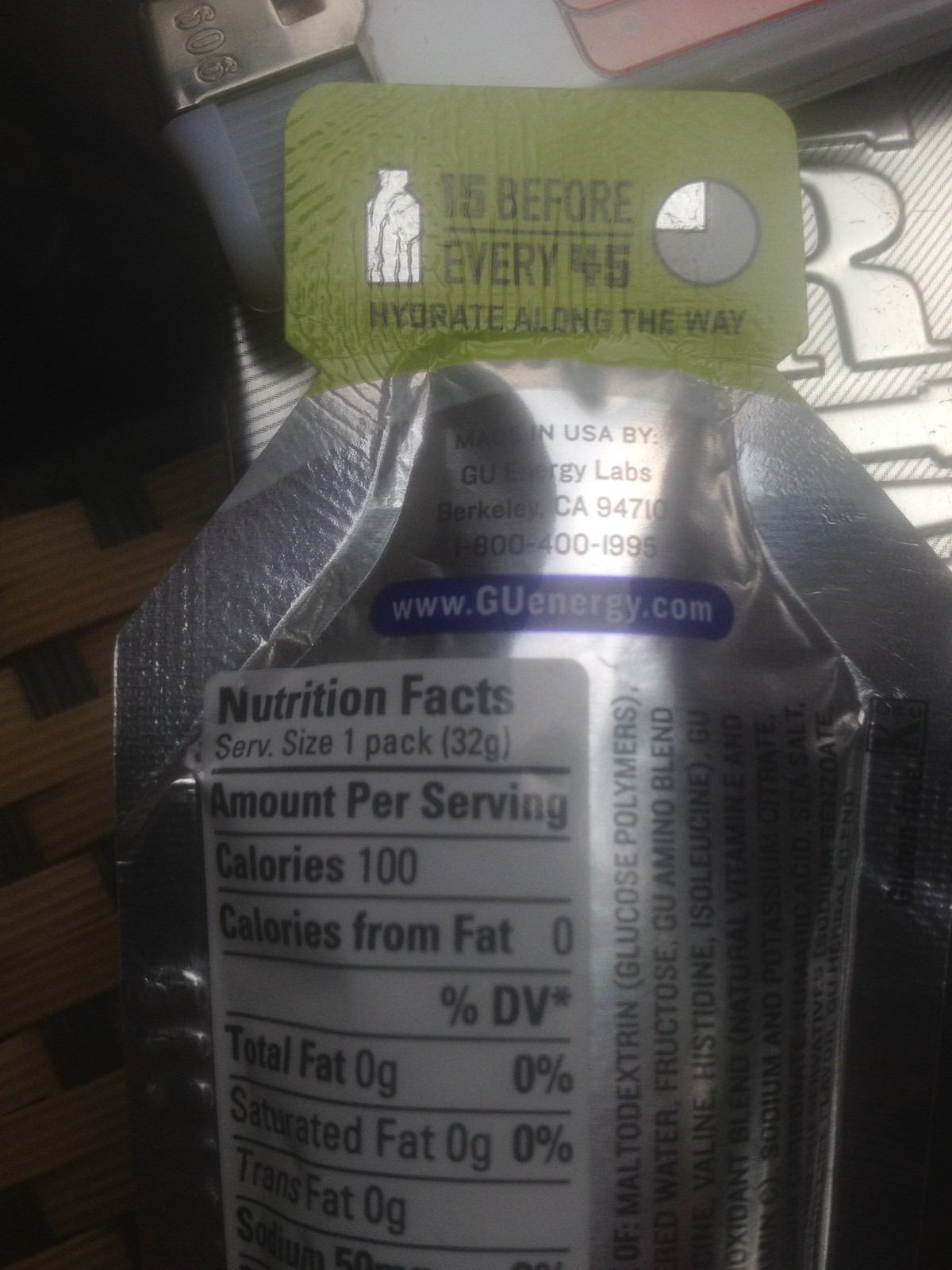This photograph is a close-up of the back of an energy gel pack designed for athletes. The packaging is a shiny, metallic silver pouch, lying on what seems to be a metallic surface, possibly a tool chest or a tabletop. At the top of the pouch, there is a green tear-off tab that reads in black text, "15 before every 45. Hydrate along the way." Flanking this message are icons: a water bottle on the left and a pie chart on the right, presented in dark gray and light gray.

Below the green tab, on the silver portion, it states, "Made in USA by GU Energy Labs, Berkeley, California 94710," followed by the contact number "1-800-400-1995" and the website "www.guenergy.com." The nutritional facts section, set within a white rectangle, details the following per serving (32 grams): 100 calories, 0 calories from fat, 0 total fat, 0 saturated fat, 0 trans fat, and 50 milligrams of sodium. Some of the ingredients listed sideways include maltodextrin, glucose polymers, filtered water, fructose, GU amino blend, valine, histidine, isoleucine, oxidized blend, natural vitamin A, sodium, and potassium citrate.

The photograph, though taken in dim lighting, highlights the glossy and reflective quality of the packaging, making its details easily discernible.